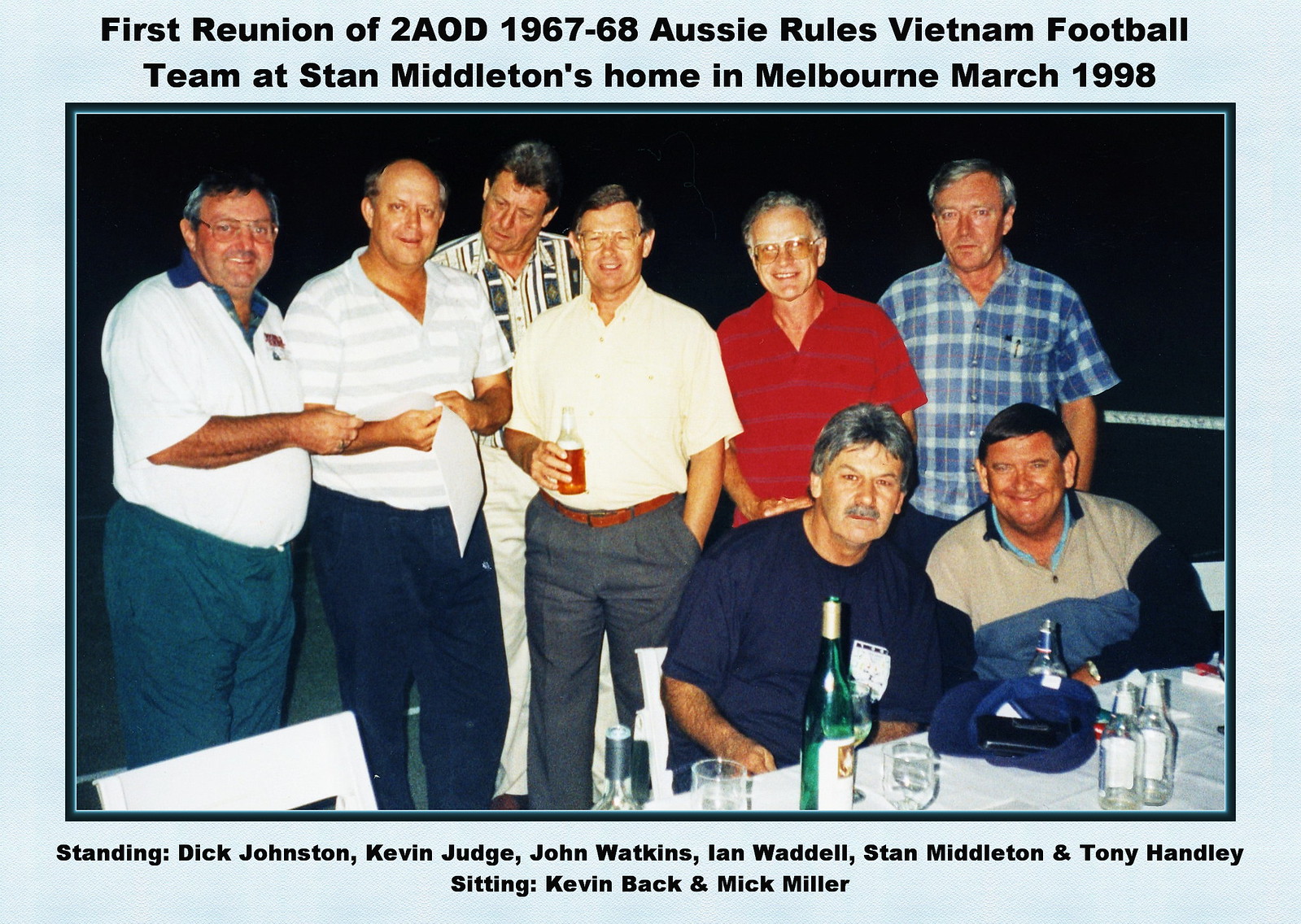This vividly detailed image captures a momentous reunion of the 2AOD 1967-68 Aussie Rules Vietnam football team, held at Stan Middleton's home in Melbourne in March 1998. Set against a light blue background with a highlighted border and textual overlays, the color photograph shows eight middle-aged, mostly gray-haired men. The scene is brightly lit by the camera flash, revealing six men standing and two sitting at a table adorned with several wine and liquor bottles and glasses. The men are casually dressed in button-down shirts with collars, smiling as they celebrate together. In the background, one gentleman holds a bottle of beer. The text at the top reads, "First reunion of 2AOD 1967-68 Aussie Rules Vietnam football team at Stan Middleton's home in Melbourne, March 1998." The bottom of the image identifies those present: Standing - Dick Johnston, Kevin Judge, John Watkins, Ian Waddell, Stan Middleton (wearing a red shirt), and Tony Handley; Sitting - Kevin Beck and Mick Miller.